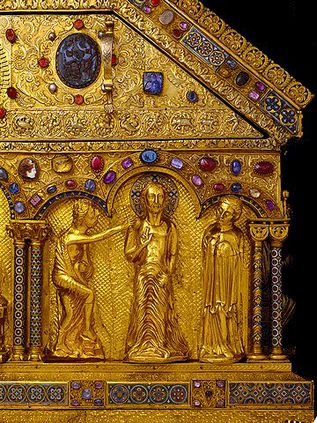This intricate bas-relief sculpture, likely an antique religious icon, depicts a central figure identified as Jesus Christ, flanked by two other figures, possibly priests or common individuals, set within an ornate, indoor setting. The entire piece appears to be crafted from solid gold, richly adorned with an array of precious jewels in hues of blue, red, amethyst, and yellow. Jesus, positioned beneath a gabled roof-like pediment embellished with jewels, is distinguished by a halo behind his head, accentuated with gold and blue tones. He gazes directly forward, raising his right hand in a gesture of blessing with his index and middle fingers extended. To Jesus' left, another robed figure extends an arm to rest a hand on Jesus' shoulder, while to his right, a similarly robed individual, adorned with a headdress, looks on in reverence. The scene is framed by decorative columns and intricate bottom trim, with all three figures standing in an archway beneath the elaborate pediment. The black background emphasizes the brilliance and detail of the gold and jewel-encrusted artwork, portraying an atmosphere of awe and sacredness.